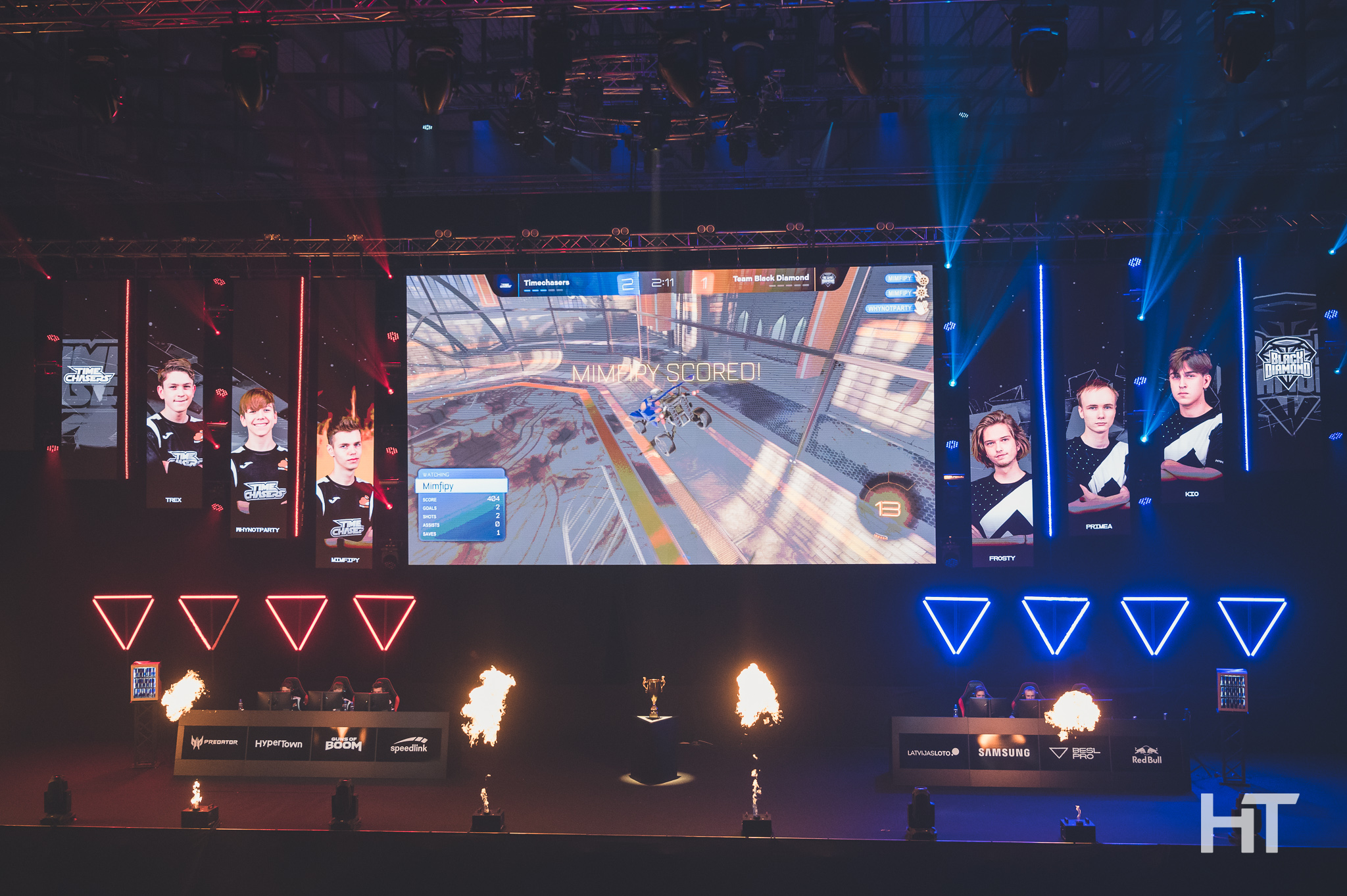The photograph captures an intense live competition on a stage set in a stadium-like venue. At the front of the stage, four chutes of fire dramatically burst upward, adding to the electrifying atmosphere. The stage features two desks on either side, where players are seated—three per side. Behind the left desk, illuminated by blue neon light, are four upside-down triangles, while behind the right desk, red neon triangles provide a contrasting backdrop.

Above each desk, ascending images of the players are prominently displayed, each player's image being either surrounded in blue or red, matching the neon lights at their desk. These likely indicate the team colors and positions. In the middle of the stage, a large central screen broadcasts the heart of the competition—what appears to be a video game, possibly involving characters maneuvering around a road on bicycles or vehicles.

The top of the stage is equipped with an extensive array of lighting and fixtures, casting rays of blue and red across the scene, enhancing the visual spectacle. The overall setup, with detailed mechanics and enthralling visuals, suggests an immersive and high-stakes live gaming event, captivating both the live audience and those viewing from afar.